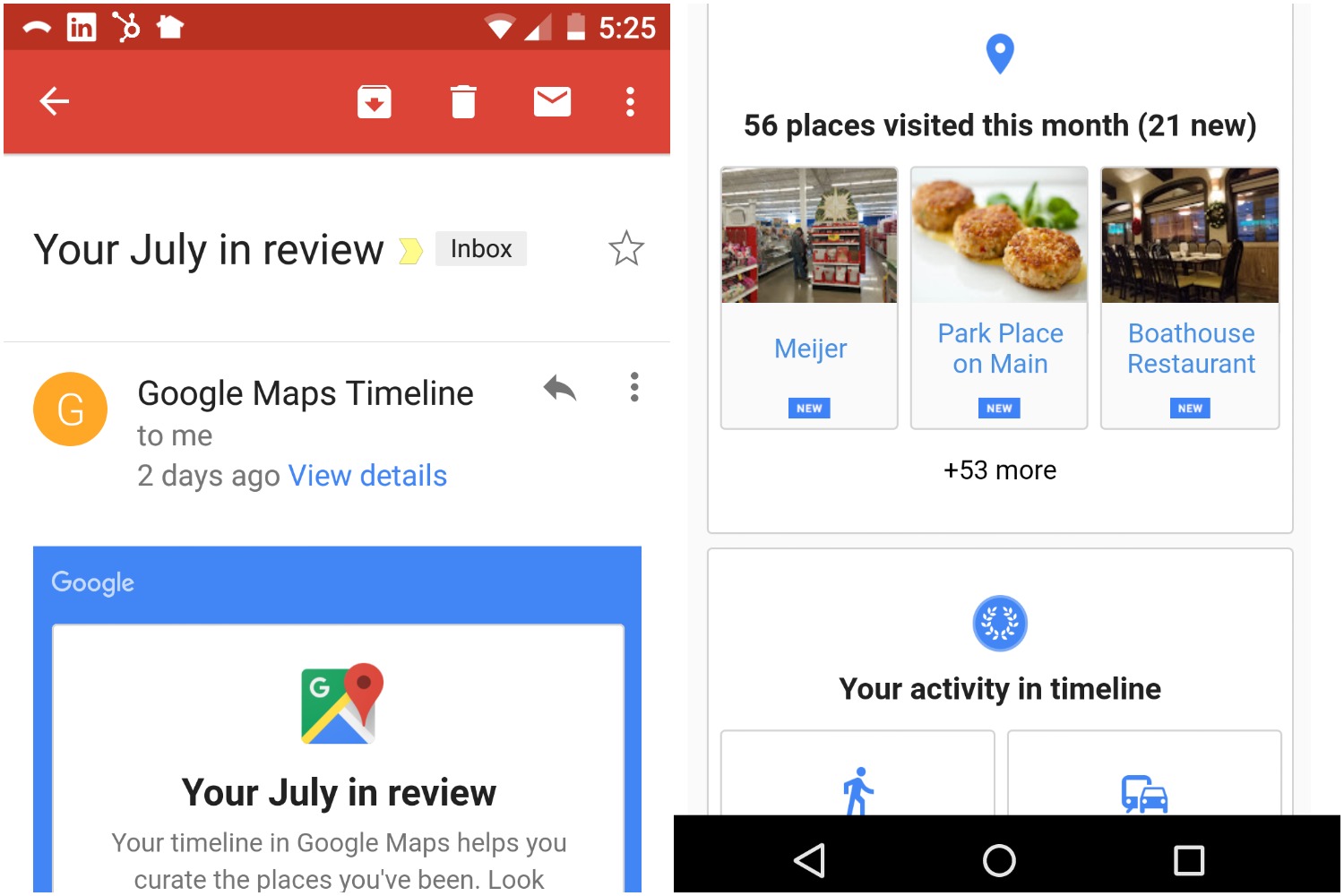The image comprises two side-by-side Google screenshots. The left screenshot is highlighted in red at the top, displaying the heading "Your July in review of Inbox." Below, there's a partial view of the Google Maps timeline, framed with a wide blue border. At the top of this blue-bordered section, "Google" is written in white, followed by the text "Your July in review: Your timeline in Google Maps helps you curate the places you've been."

In the right screenshot, the caption notes that 56 places were visited in the month, with 21 being new. The image displays three photos labeled "Mayhair," presumably a store, followed by "Park Place on Main" and another with three items resembling burgers. Additionally, the "Boathouse Restaurant" is listed under new places visited, along with a mention of "53 more." Below these entries, there's an activity timeline, and at the bottom of the image is a black bar.